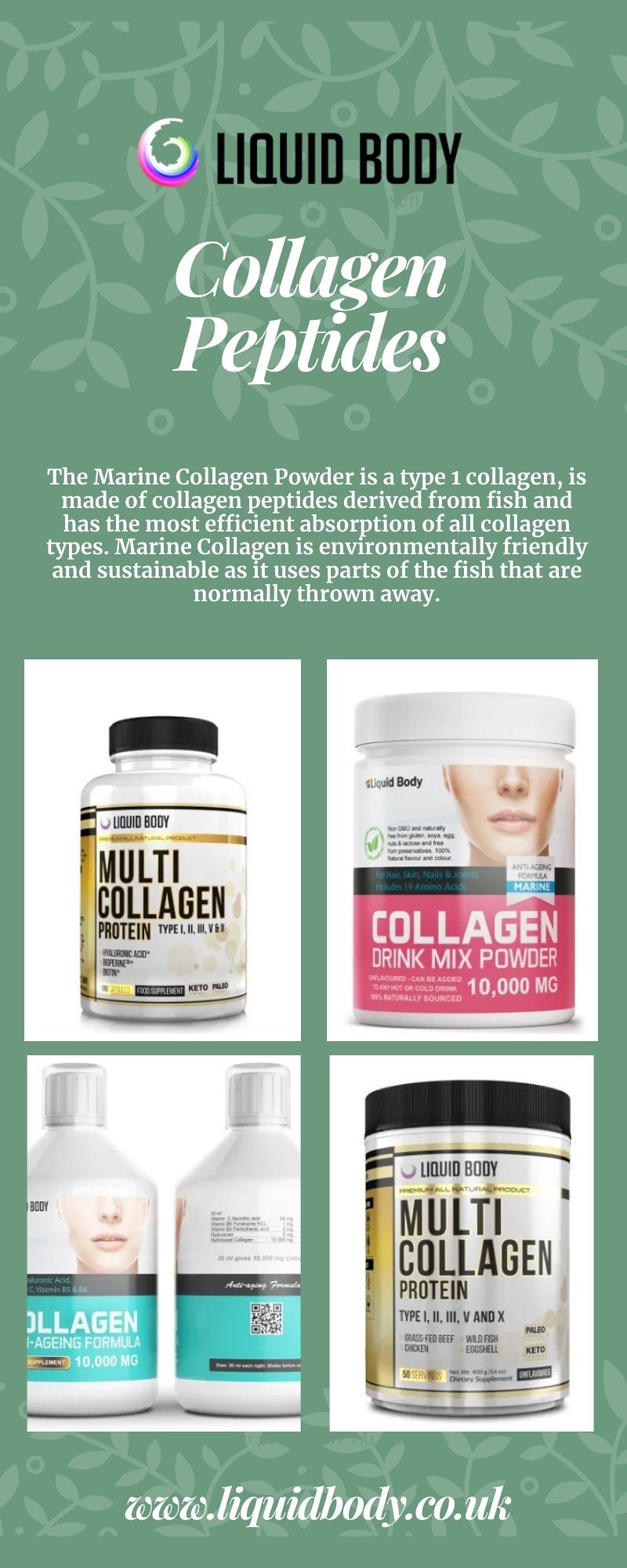This is a detailed advertisement for Liquid Body Collagen Peptides, set against a light green background adorned with leafy patterns. At the top, the brand name "Liquid Body" is prominently displayed in black lettering, followed by "Collagen Peptides" in white font. Beneath this, in smaller white text, it reads: "The Marine Collagen Powder is a type 1 collagen, made of collagen peptides derived from fish and boasts the most efficient absorption of all collagen types. Marine collagen is environmentally friendly and sustainable as it utilizes parts of the fish that are typically discarded."

The bottom half of the page features a 2x2 grid with four product images. The first image is of a bottle labeled "Liquid Body Multi-Collagen Protein." Adjacent to it is a "Liquid Body Collagen Drink Mix Powder" container. Below these, on the left, is an anti-aging formula featuring a woman's face, while to the right, there are two smaller bottles of pre-mixed collagen drink. The ad concludes with the brand's website, www.liquidbody.co.uk, in white font at the bottom.